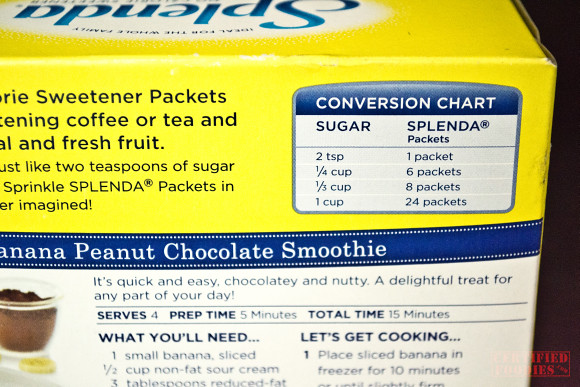This close-up photograph captures the back of a Splenda sweetener packets box. The majority of the image is taken up by the bright yellow upper half of the box, which features the Splenda logo in blue text on a white oval. The logo appears slightly cut off and is positioned towards the top center. The lower portion of the box transitions to white and contains various informational elements.

Towards the upper right, there's a detailed sugar-to-Splenda conversion chart outlined with a blue border and white background. The chart lists conversions such as two teaspoons of sugar to one Splenda packet, one-fourth cup of sugar to six packets, one-third cup to eight packets, and one cup to 24 packets. Additional text in black on the left side of the chart explains, "Sweetener packets for coffee or tea and real fresh fruit."

Lower on the box, a recipe for a Banana Peanut Chocolate Smoothie is displayed, emphasizing its quick, easy preparation and delightful chocolatey, nutty flavor. The recipe section is predominantly white, with blue text detailing the ingredients: "one small sliced banana, half a cup of nonfat sour cream, three tablespoons reduced-fat..." and steps like, "place sliced banana in freezer for 10 minutes." The smoothie ingredients are pictured, including a clear bowl with brown powder, a piece of chocolate, and a slim banana slice.

A blue ribbon wrapped around the middle visually divides the yellow and white portions of the box. There’s also a partially visible red stamp in the bottom right corner, which appears to say "classified" in a red-rimmed box, although some of the text is obscured.

Overall, the image focuses tightly on the detailed components of the packaging, providing a clear view of the brand, important conversion information, and the enticing smoothie recipe.